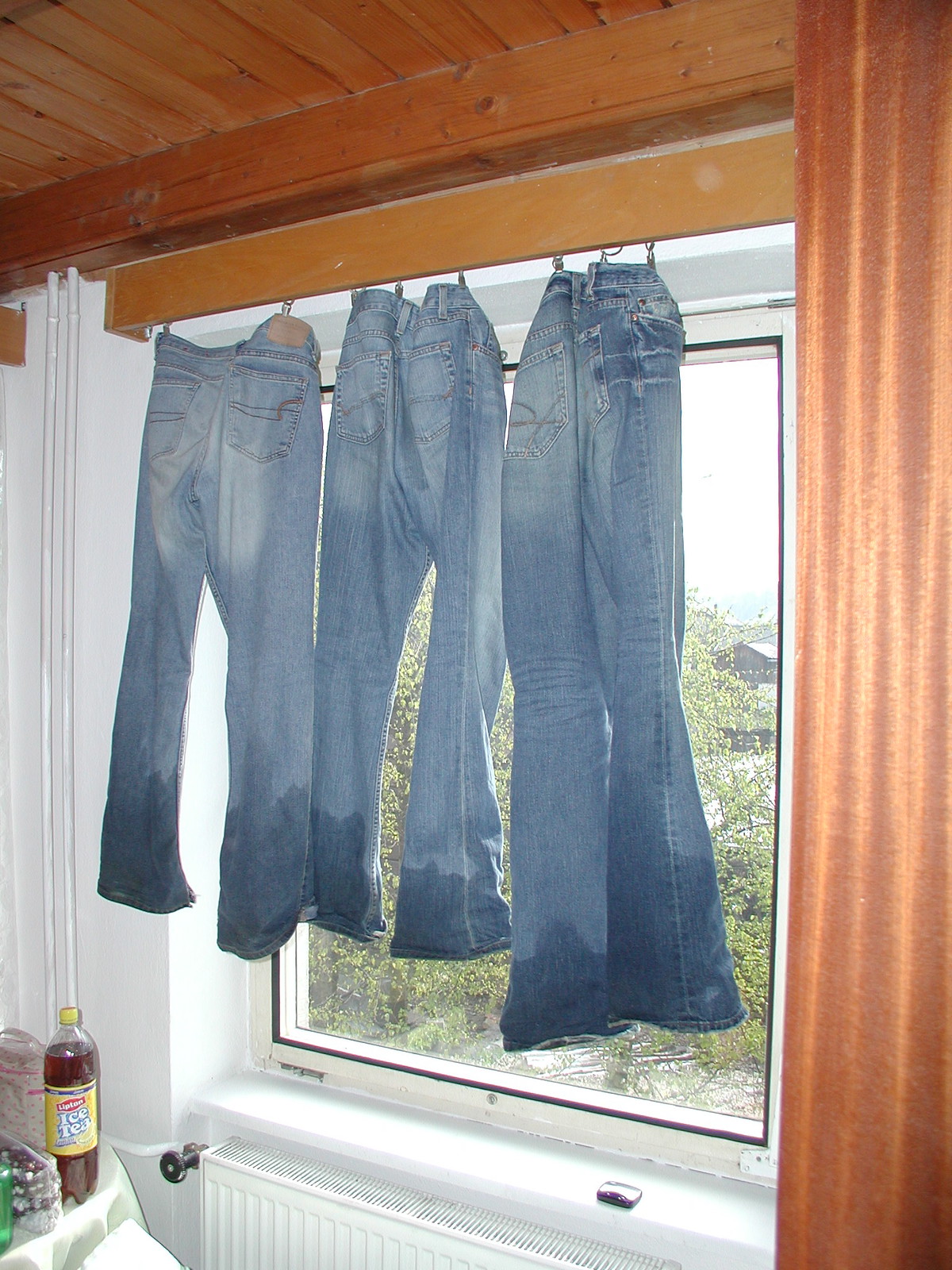In a black and white photograph, three pairs of blue jeans, appearing to be wet at the bottom, are hung up by their belt loops in front of a window, possibly with alligator clasp-type metal hangers. The jeans, varying in length, dangle down in front of an open window within a wooden-framed house. The window, framed in a white or redwood-ish color, overlooks a garden with green trees and possibly a brown barn in the background. Beneath the jeans is a heating radiator or furnace. White curtains frame the window, while above, a slatted wooden ceiling can be seen. In the bottom left of the image, a small table holds a bottle of Lipton's iced tea and an indistinct green object.